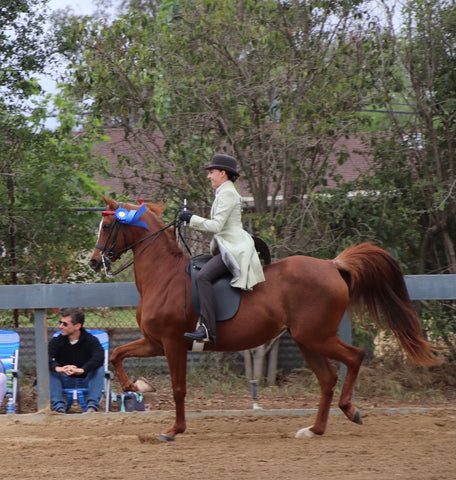This is a photograph taken at an outdoor horse show, showcasing a woman jockey riding a reddish-brown horse in a dirt arena. The horse, adorned with a black bridle and a blue ribbon on its head, has one front hoof and one hind hoof raised as if in mid-step, giving the impression of motion. The horse's thick, full tail is light brown at the base, transitions to dark brown, and returns to a lighter brown at the tips. The rider, a woman with short black hair at chin length, is wearing a beige long jacket that is open at the bottom, gray flared pants, black boots, and black gloves. Her boots are in metal stirrups, and she holds the black reins firmly. She accessorizes with a brown bowler hat atop her head.

In the background, there is a spectator, a white man with short black hair, dressed in a black jacket and blue jeans, sitting in a blue beach chair and wearing sunglasses while looking off to the left. He is positioned near a blue wooden fence with a metal chain-link fence underneath. Beyond the fences, the scene blurs into trees, power lines, and the roof of a brown house.